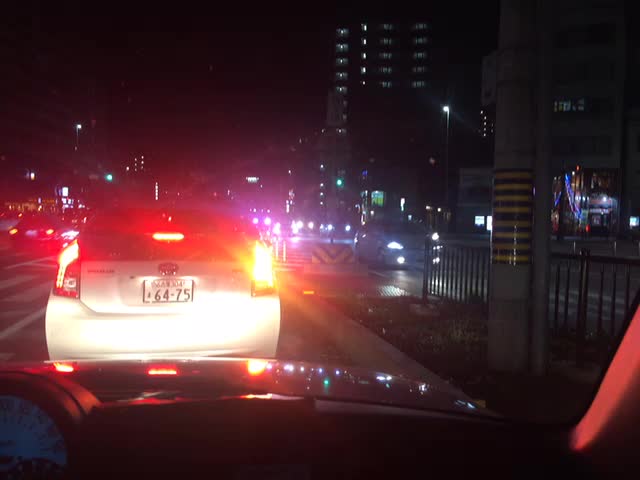A nighttime cityscape as seen from inside a car, possibly from the passenger seat, captures the urban vibrance through the windshield. The sky is an uninterrupted expanse of black, devoid of stars or any gradient, underscoring the late hour. Glimpses of tall buildings with sporadically lit windows suggest a modest urban setting, not overly dense but distinctly metropolitan. The car's dashboard frames the bottom of the scene, anchoring the view within the vehicle. Ahead, the silhouette of a white car leads the way, while another vehicle appears parked on the side of the street. Further in the distance, a few street and traffic lights punctuate the darkened environment, casting a subtle glow on the pathway ahead. The image conveys the quiet yet persistent pulse of city life at night.